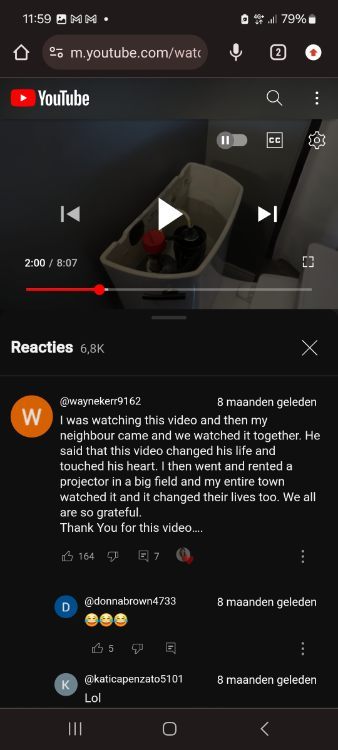This mobile screenshot captures a YouTube page accessed via the web browser on an Android device, identifiable by the URL "m.youtube.com" in the navigation bar, indicating the mobile version of the site. The top bar reveals the device's current time as 11:59, potentially following a 24-hour format, which aligns with the German language text displayed within the YouTube interface.

Status icons at the top of the screen indicate a saved image, two Gmail notifications, a notification dot, charging status, mobile data, 79% battery, and a three-bar signal strength. The navigation bar features the home button, URL "YouTube.com," a voice button (microphone symbol), two browser tabs, and a red arrow within a white circle, possibly an upload button. The familiar YouTube logo is also visible.

A paused video is displayed two minutes into an 8:07 duration. Beneath the video, comments are featured, beginning with Reactees 6.8k, followed by a comment from Waynecker9162. The comment elaborately details the impact of the video, mentioning the viewer's experience watching it with a neighbor, renting a projector to show it in a field, and how it purportedly transformed the entire town's life—a narrative that seems facetious due to subsequent comments containing laughing emojis and a simple "LOL."